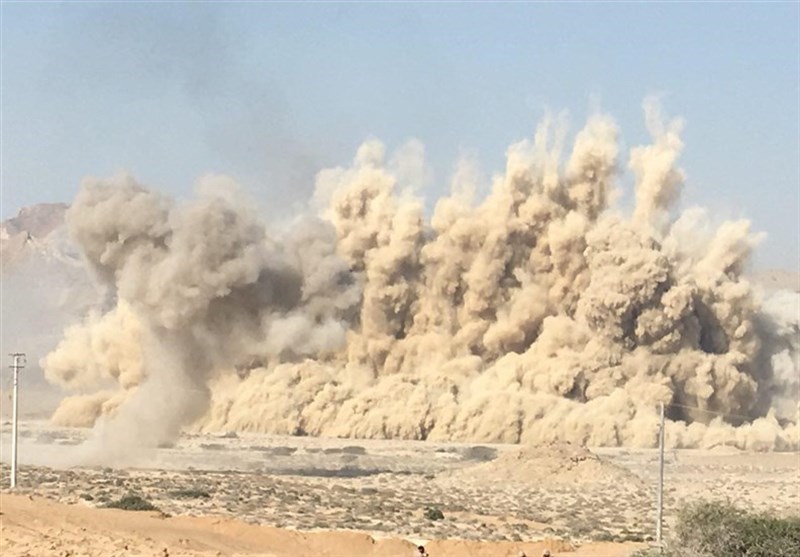This is a color photograph capturing what appears to be a significant explosion or dust storm in an arid, desert-like landscape. The image is dominated by a towering cloud of brown dust or smoke, with smaller sections displaying different shades of brown and lighter colors. The dust cloud takes up most of the frame, with a very rocky and flat landscape visible past the explosion. There is a bluish-gray sky above, devoid of any clouds. In the background, some black smoke can be seen rising. A telephone pole stands to the far left, along with two white power lines slicing through the scene. Though the ground appears barren with no visible people, animals, structures, or vehicles, there's a faint silhouette of what looks like a tree and possibly a stone-walled bridge or road in the distance. The source of the explosion or dust storm remains unidentified.